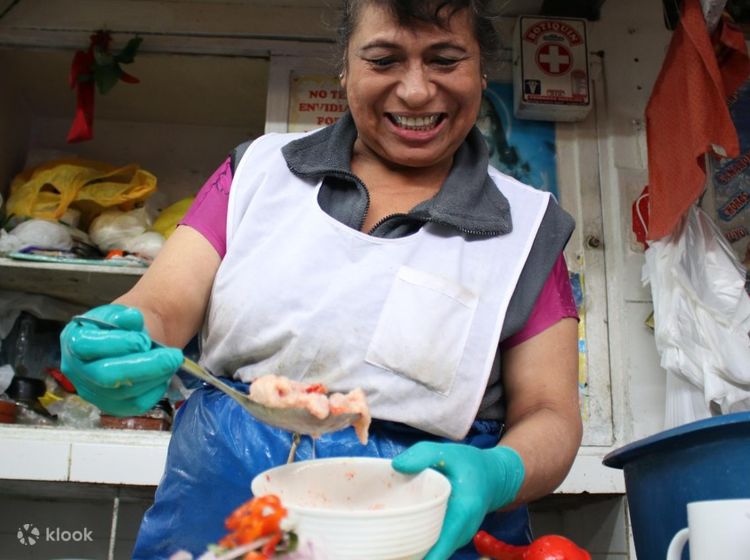The photograph features a smiling, middle-aged woman with brown skin and her hair pulled back into a ponytail, showcasing her wide, toothy grin. She holds a large ladle or spoon and a white bowl filled with lumpy, gumbo-like soup, faintly pinkish in color. Dressed in a layered outfit, she sports a purple short-sleeve shirt beneath a black or blue vest, topped with a white apron tied around her waist. Additionally, she has wrapped a blue tarp-like material around her waist, likely for extra protection. She is also wearing light blue latex gloves. Positioned at a leaning angle, she stands in what seems to be a cluttered and slightly dirty kitchen or indoor space, discernible by the old, white painted wooden cabinets and assorted items, including fabric piles and plastic bags on the shelves behind her. The image appears to be an impromptu snapshot, capturing her in a moment of cooking or serving food, radiating happiness and fulfillment.